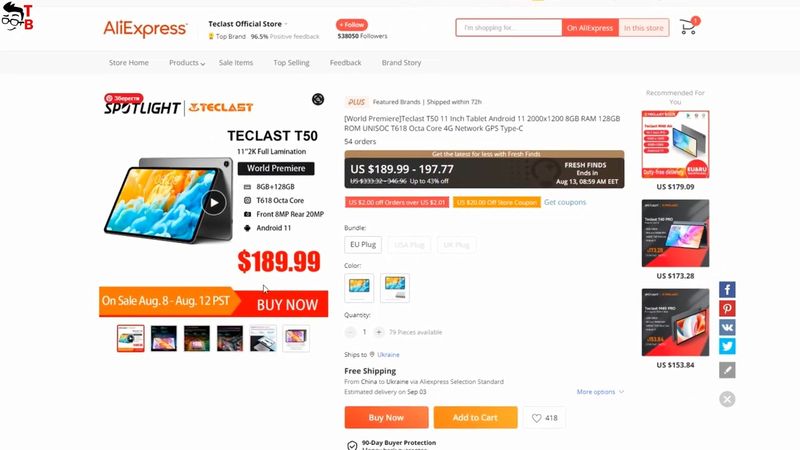The screenshot captures a product listing on the AliExpress website, evidenced by the signature red "AliExpress" logo situated in the upper left corner against a white background. Adjacent to the logo is a small, schematic drawing resembling a man's head, adorned with hair, glasses, eyebrows, and a simplistic smile. Accompanying this illustration are the red letters "T" and "B" stacked vertically underneath.

In the header section, the text "10-Class Official Store" designates the specific AliExpress vendor. The featured product, prominently displayed on the left side of the screen, is labeled as the Tech Class T50, which appears to be a smartphone.

The smartphone's screen showcases an artistic display, split between blue clouds on the upper half and yellow clouds on the lower half. The price for this device is prominently shown in red, listed at $189.99.